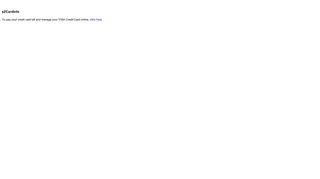The screenshot captures a largely blank, white webpage, giving an impression of minimal content. At the top, there are two distinct lines of text. The upper line features a single word in bold, black text with no spaces, making it appear compressed. Beneath this bold header, a sentence is displayed in a smaller font, but it's too tiny to be read clearly, possibly due to the zoom level of the image. The overall aesthetic suggests a clean but underdeveloped or placeholder page.